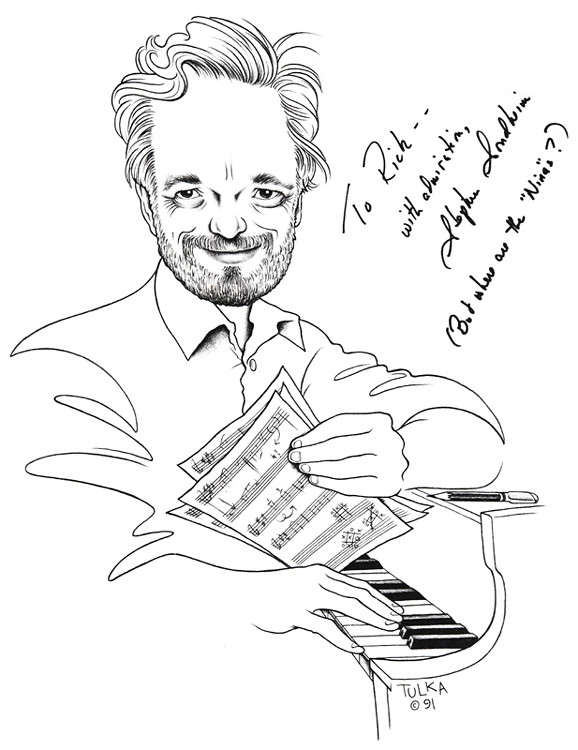This black and white sketch, likely done with black ink or marker, portrays a white male from the waist up, seated at a piano. The man has a distinctive appearance characterized by a large, square-shaped forehead, wavy hair that moves upwards and towards the left, and a thin beard and mustache, with some beard stubble. His expression features a closed-mouth smile, with noticeable wrinkles around his cheeks and crow’s feet by his eyes. He wears a button-up collared shirt. His left arm rests atop the piano, holding a couple of sheets of music, while his right hand is positioned on the piano keys, although only the interior part of the arm is visible.

The piano itself shows black and white keys at the bottom right of the image, with a pencil lying on its surface near the man's left elbow. There is diagonal writing at the top of the image that reads: "Too Rich with admiration," followed by an illegible cursive signature. At the bottom, there's additional text, also in cursive, which says "Alfie," and then in parentheses, "but where are the Nina's?"